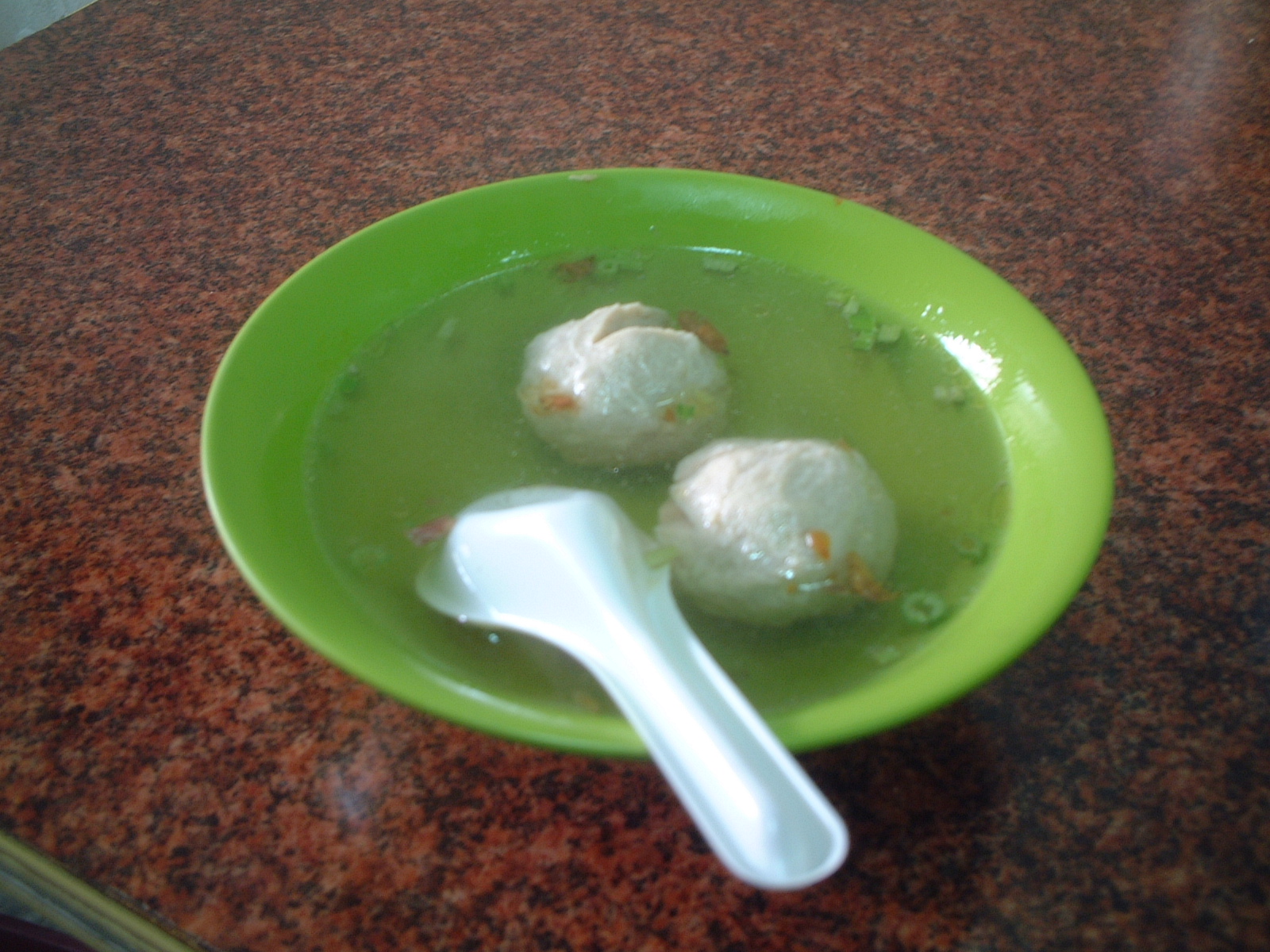In this photograph, a green ceramic bowl is prominently displayed on a brown and black granite kitchen counter, showcasing a captivating mix of elements. The counter features intricate dot patterns in various shades of brown, lending an aesthetically pleasing backdrop. Inside the bowl, there is a clear liquid, possibly a soup, accompanied by two round, white edible items, likely matzo balls, sitting serenely in the broth. Floating in the liquid are small, colorful pieces, most notably green, and a few orange ones, reminiscent of fruit loops. A white spoon, possibly ceramic, is placed inside the bowl, adding to the overall composition. The image offers a harmonious blend of colors and textures, capturing a simple yet intriguing culinary scene.